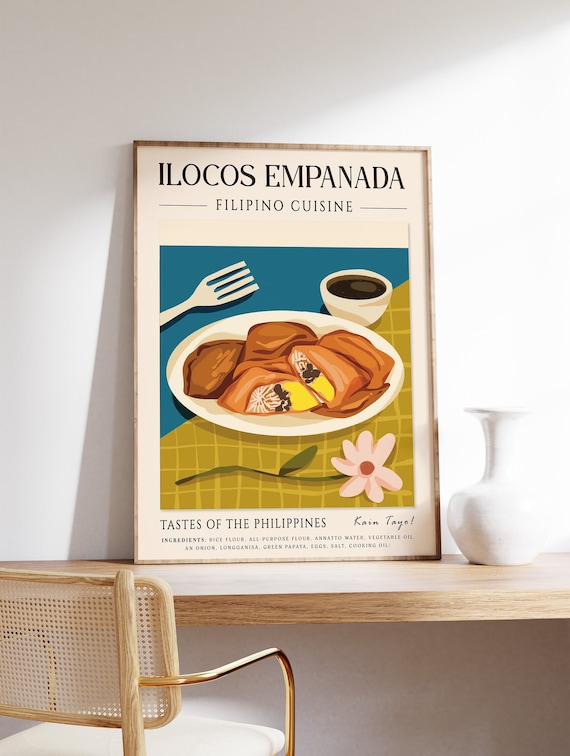The image captures a wooden table with a laminate finish, holding a white vase with a slim neck and a flat, rounded base. Positioned against a white wall, there is a framed poster prominently displaying "Ilocos Empanada, Filipino Cuisine." Below the text, the poster features an illustration divided diagonally: the top left in dark blue and the bottom right in yellow with white grid lines. At the center of the illustration, a white plate holds four pieces of food with yellow centers, accompanied by a fork above, a pink flower with a green stem beneath, and a cup of coffee to the side. The brass-armrested, mesh-backed wooden chair sits tucked under the table. Overall, the scene suggests a tastefully arranged spot, possibly in a Filipino eatery or café, emphasizing the inviting and colorful presentation of traditional cuisine.